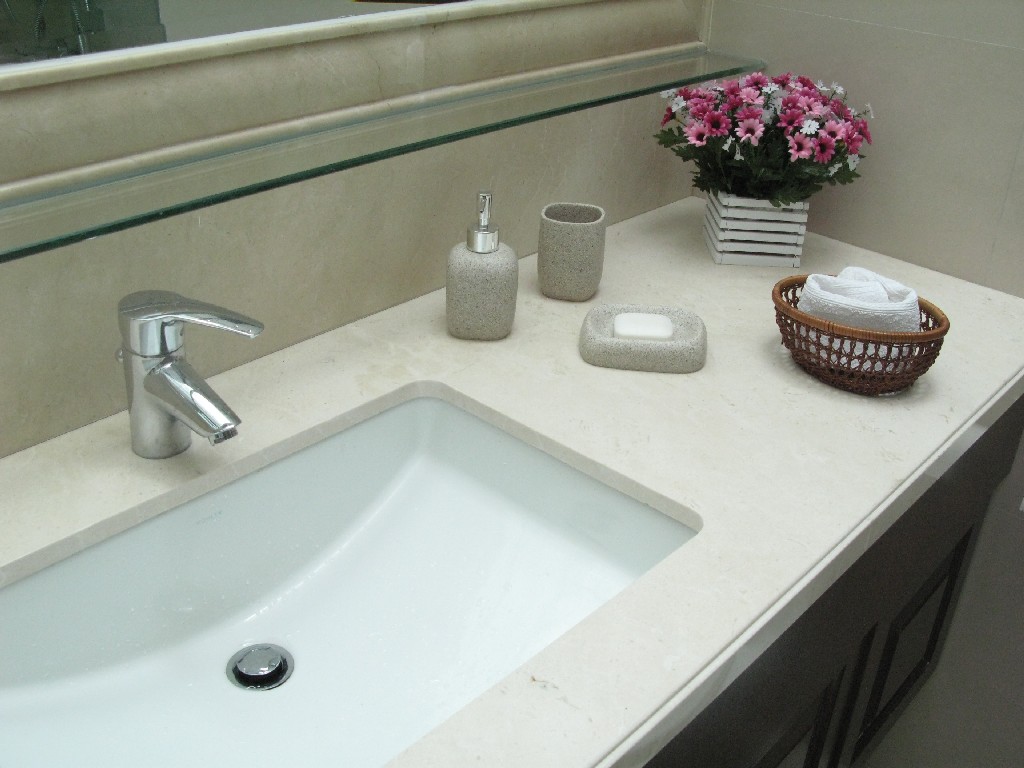The image showcases a pristine and well-organized bathroom washbasin area with a working surface to its right. The surface is clean, white, and offers a minimalistic yet elegant appearance. The sink features a push-up, push-down seal, adding a sleek touch to its functionality. Below the countertop, there is a cupboard finished in a very dark grey, creating a striking contrast with the paler elements of the scene.

The bathroom wall is a soothing pale grey color, while the splashback behind the sink is a very light sage green with a subtle green stripe, adding a hint of color without overwhelming the space. Above the washbasin, a mirror is partially visible, hinting at a larger reflective surface that likely adds depth and utility to the room.

On the white countertop, there is a medium grey pump-action hand wash dispenser and a matching dish of soap, maintaining the clean and cohesive color scheme. A small, oval rattan or wicker basket holds a neatly folded, clean white towel. This handmade, open-weave basket adds a touch of rustic charm to the modern setting.

At the back of the countertop stands a white, square vase or plant holder with five black stripes encircling it. Nestled within are vibrant, primarily pink flowers with green leaves and a few small white blooms. The flowers resemble daisies, with varying shades of pink, from dark to pale, adding a fresh and lively element to the arrangement.

To the right of the hand wash dispenser, there is an empty toothbrush holder, contributing to the tidy and uncluttered look of the area. The overall setup exudes a warm and inviting ambiance, suggesting it might be part of a well-maintained hotel room. The combination of cleanliness, thoughtful details, and pops of color makes the washbasin area both functional and aesthetically pleasing.